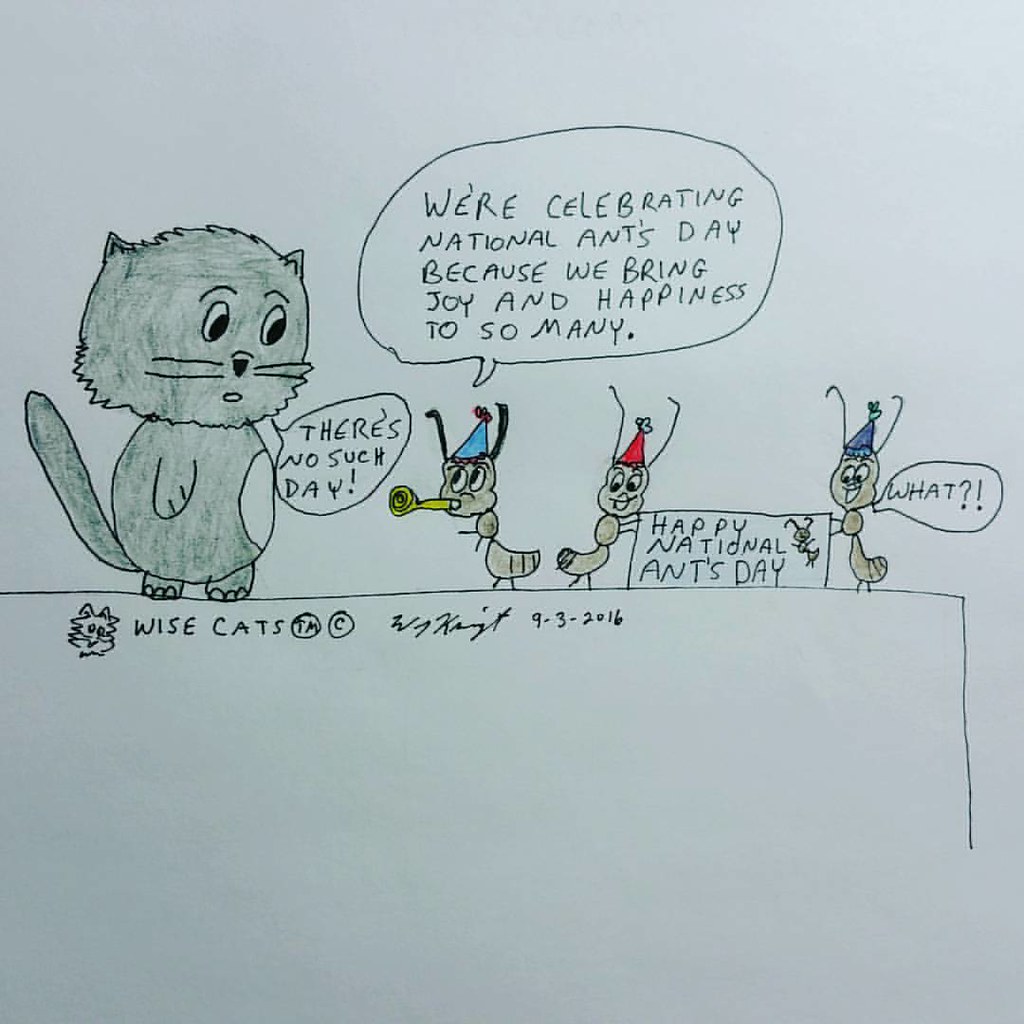The image is a colorful cartoon drawing featuring anthropomorphic animals. The main characters are a gray cat standing upright and three ants with party hats, celebrating on a raised platform. The ants are hosting a "Happy National Ant Day" party, marked by a bright banner held by two ants. One ant, positioned on the left and blowing a party noisemaker, exclaims, "We're celebrating National Ants Day because we bring joy and happiness to so many." The gray cat skeptically replies, "There's no such way." Meanwhile, the ant on the far right responds with a surprised "What?" Text elements in the image include a "Wise Cats™ ©" label, the artist's signature, and the date "9-3-2016."